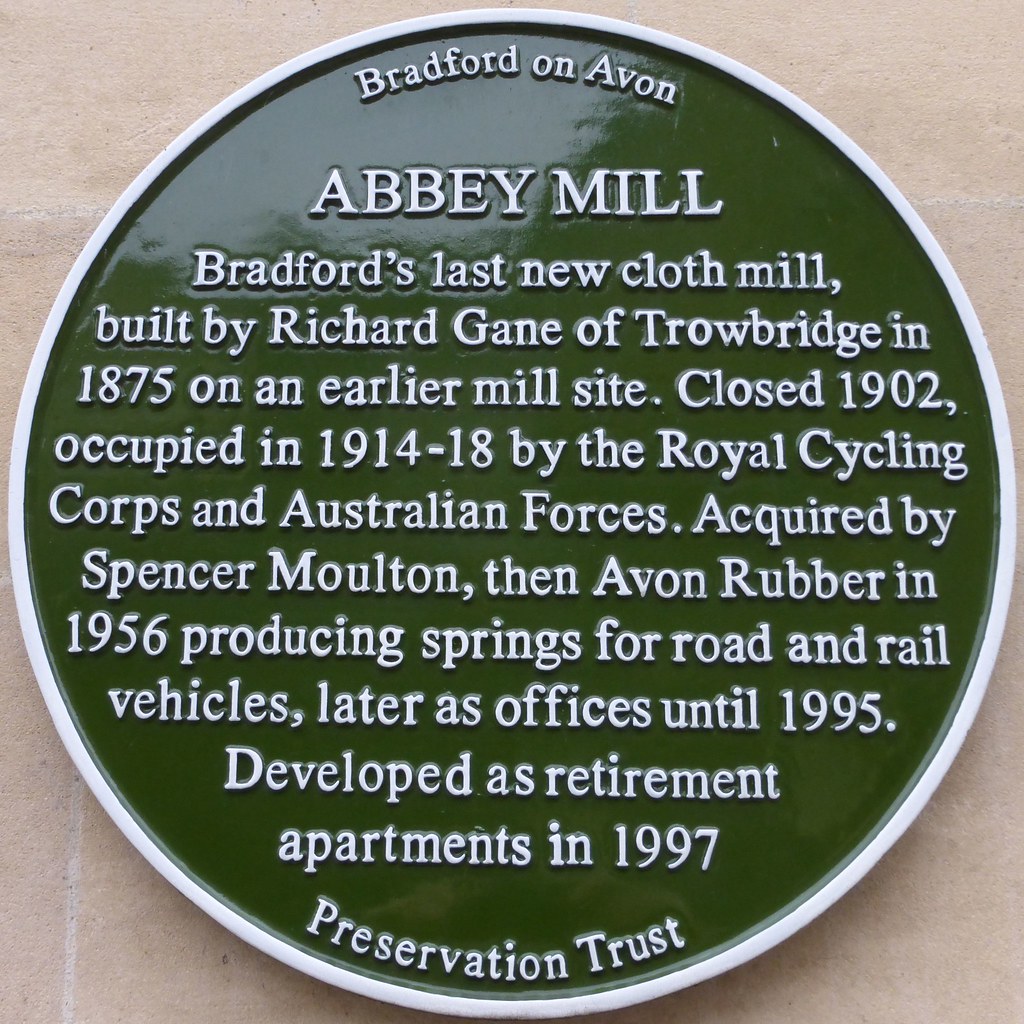The image showcases a historical plaque from Bradford-on-Avon against either a peach or beige-colored background that might be a concrete wall. The plaque, circular in shape, features a dark green to black background with a distinct white or silvery rim and raised white lettering. The plaque's inscription provides detailed historical information: "Bradford on Avon, Abbey Mill, Bradford's last new cloth mill, built by Richard Gain of Trowbridge in 1875 on an earlier mill site. Closed 1902, occupied in 1914-18 by the Royal Cycling Corps and Australian forces. Acquired by Spencer Moulton, then Avon Rubber in 1956, producing springs for road and rail vehicles, later used as offices until 1995. Developed as retirement apartments in 1997. Preservation Trust." This sign highlights the rich history of Abbey Mill, its various uses over time, and its modern transformation into retirement apartments.